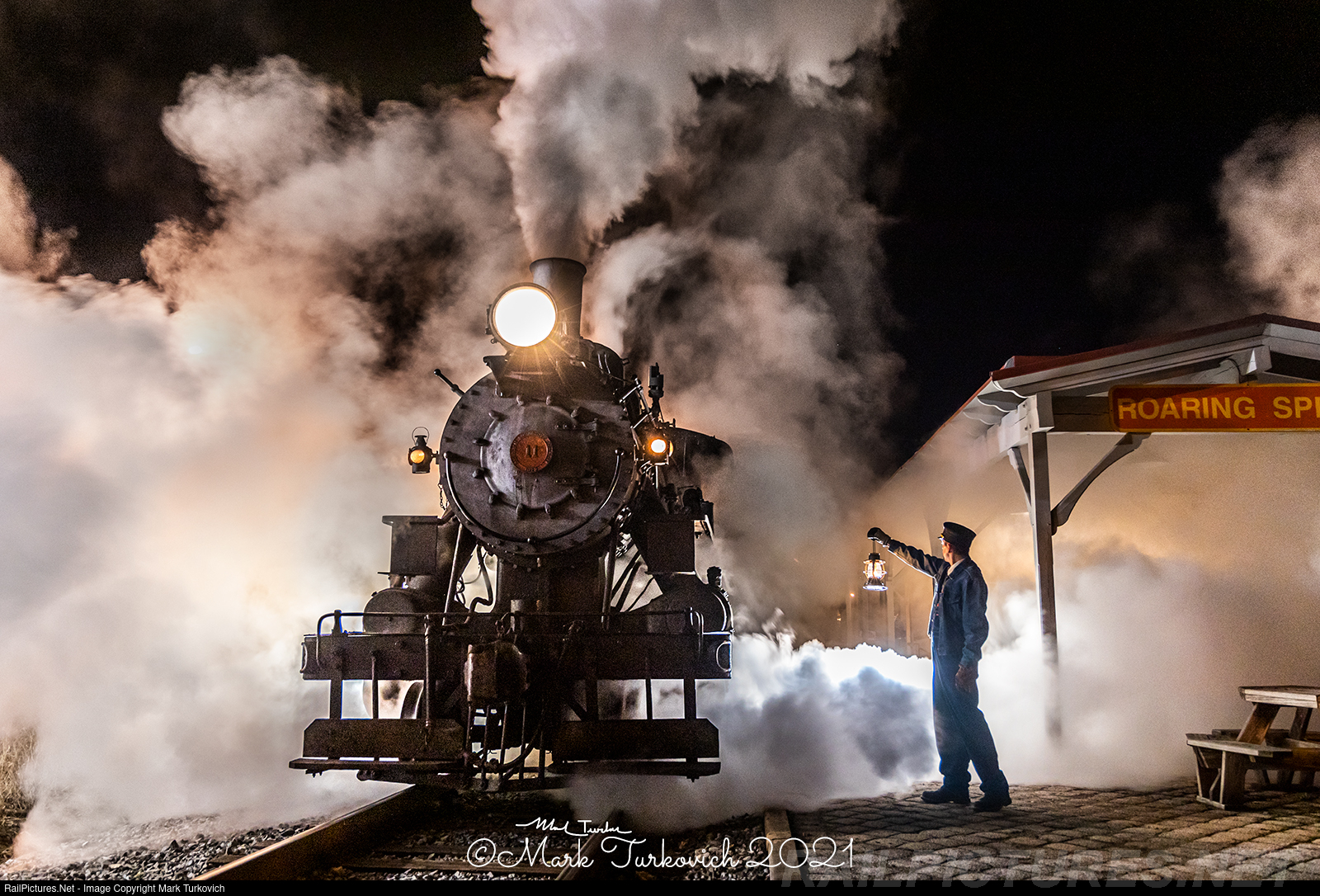This atmospheric, professionally crafted illustration by Mark Turkovich (2021) captures an evocative nighttime scene of a steam engine pulling into a station. The forefront of the train features a bright headlight shining towards the viewer, flanked by two yellow lights and a red logo at the center. Billowing gray, dark, misty steam envelops the surroundings, obscuring many details and imbuing the image with a sense of mystique. An engineer, dressed in a navy blue suit, stands to the side holding a lantern, looking away from the viewer. A station with a sign that reads "Roaring Springs" and a small picnic bench-like object are partially visible through the dense steam. The scene is further accentuated by a black sky, adding to the historic ambiance reminiscent of the 1800s. Mark Turkovich's signature and copyright are placed prominently at the bottom, along with some white text on a black border.